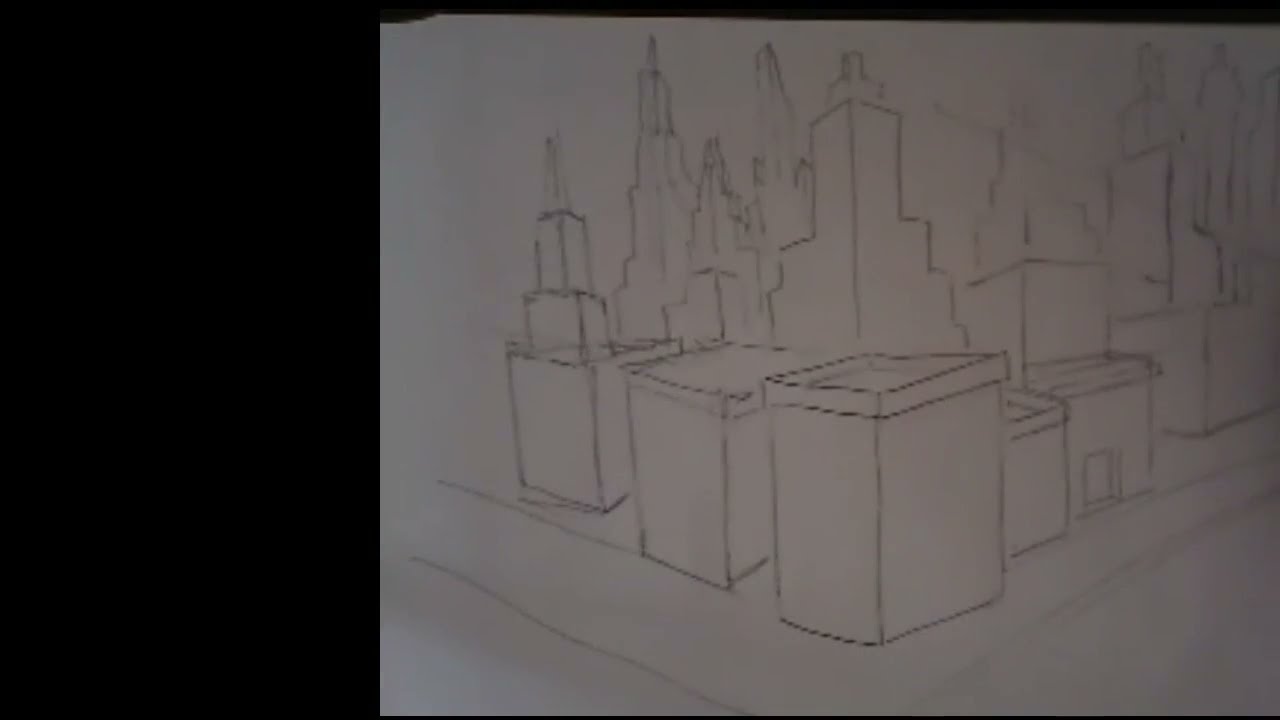This image, likely a screenshot from a video, showcases the intricate process of an artist inking a detailed cityscape sketch. The paper, positioned on the right side against a black background, displays an elaborate pencil outline featuring various buildings, including skyscrapers, shorter commercial spaces, residential apartments, and notable structures like a church with a clock tower and a water tower on a rooftop. The artist's right hand is seen holding a black ink pen, meticulously reinforcing the pencil outlines with darker, permanent lines. The pen is currently outlining an area resembling the shape of a '7,' connecting directly to the inking process. The sketch reveals a bustling urban environment reminiscent of New York City, complete with diverse rooftops, spiked and flat, and distinct architectural elements defining the cityscape.